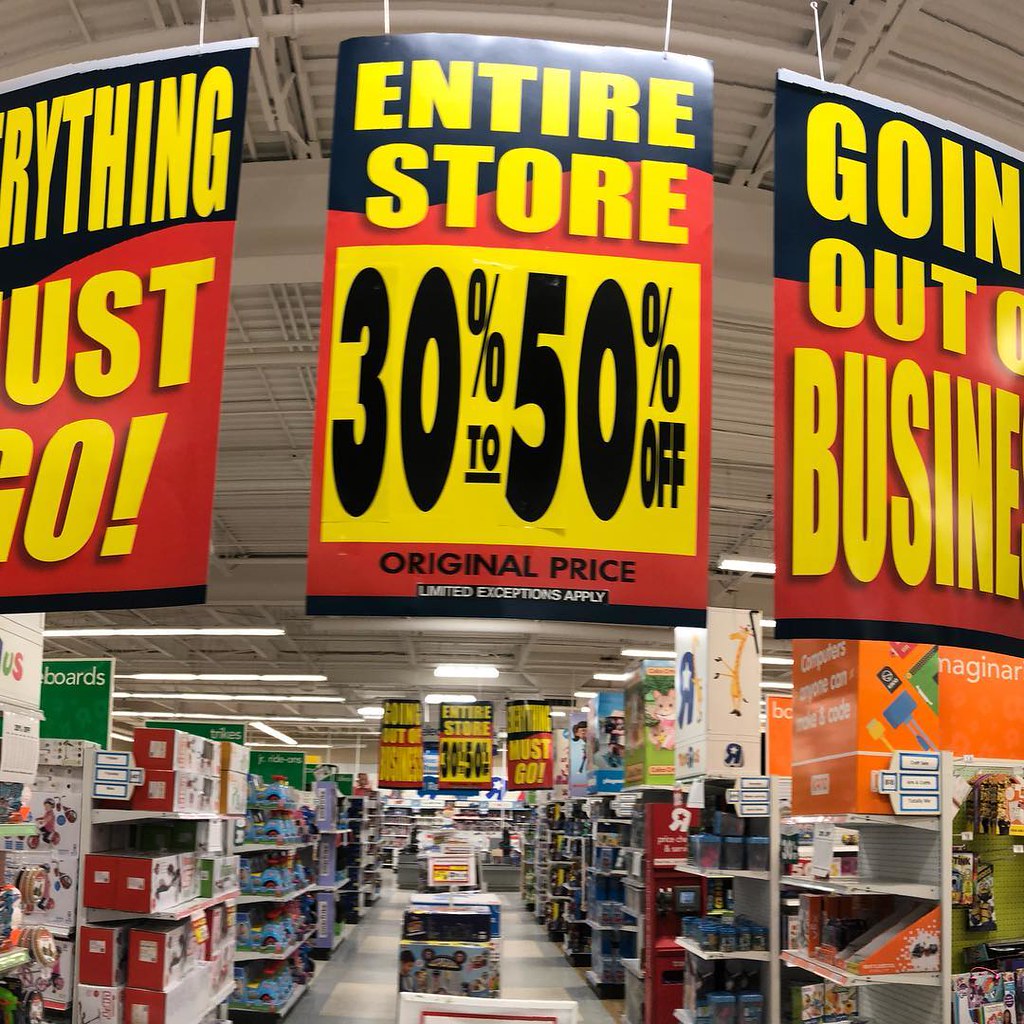This photograph depicts the interior of a Toys R Us store that is going out of business. The store features a ceiling of light gray metallic scaffolding with several long, white fluorescent lights and horizontal vent lines. The floor is tiled in light gray and off-white. A number of aisles with white shelves filled with toys and various products are visible, some of which are positioned at the end caps, which are marked with blue and white directional boxes indicating the contents of each shelf. Hanging from the ceiling are large, bright red, yellow, and black signs positioned to the left, center, and right. These signs announce "Everything Must Go," "Entire Store 30% to 50% Off, Original Price, Limited Exceptions Apply," and "Going Out of Business." The familiar Toys R Us logo and Jeffrey the Giraffe are also visible in the top right corner, emphasizing the store's impending closure.